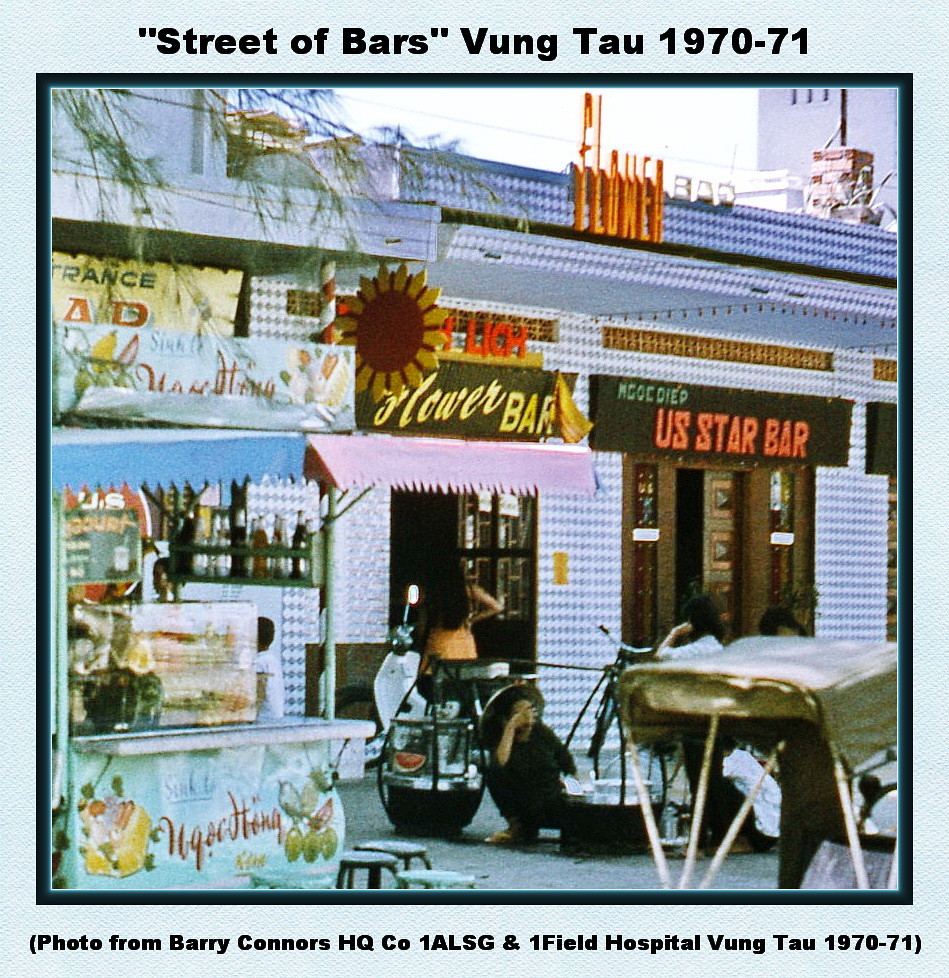This is a historic, digitally-manipulated, and framed vintage photograph titled "Street of Bars, Vung Tau, 1970-71." The frame is a dark navy blue featuring a white computer-generated matte board. Below the photograph, a caption reads: "Photo from Barry Connors, HQ CO 1 ALSG at One Field Hospital, Vung Tau 1970-71."

The image depicts two adjacent bars with quaint, old-fashioned signs: the "Flower Bar" and the "U.S. Star Bar," the latter with orange lettering. The Flower Bar building has flowers adorning it and a brown door, with a pink awning overhead. 

In front of the bars, there is an outdoor drink stand where liquor can be purchased. Several bicycles are parked along the sidewalk, and a few stools are provided for seating. A person sits on the ground, possibly taking a break, and appears to be wiping their eyes while holding their head near a kettle. Additionally, a girl with long dark hair is seen walking into one of the bars.

A palm tree's leaves partly frame the picture from the left side, and a chimney is visible atop one of the buildings. The scene, captured during the day, primarily shows workers rather than customers, giving a sense of daily life in Vung Tau during the early 1970s.